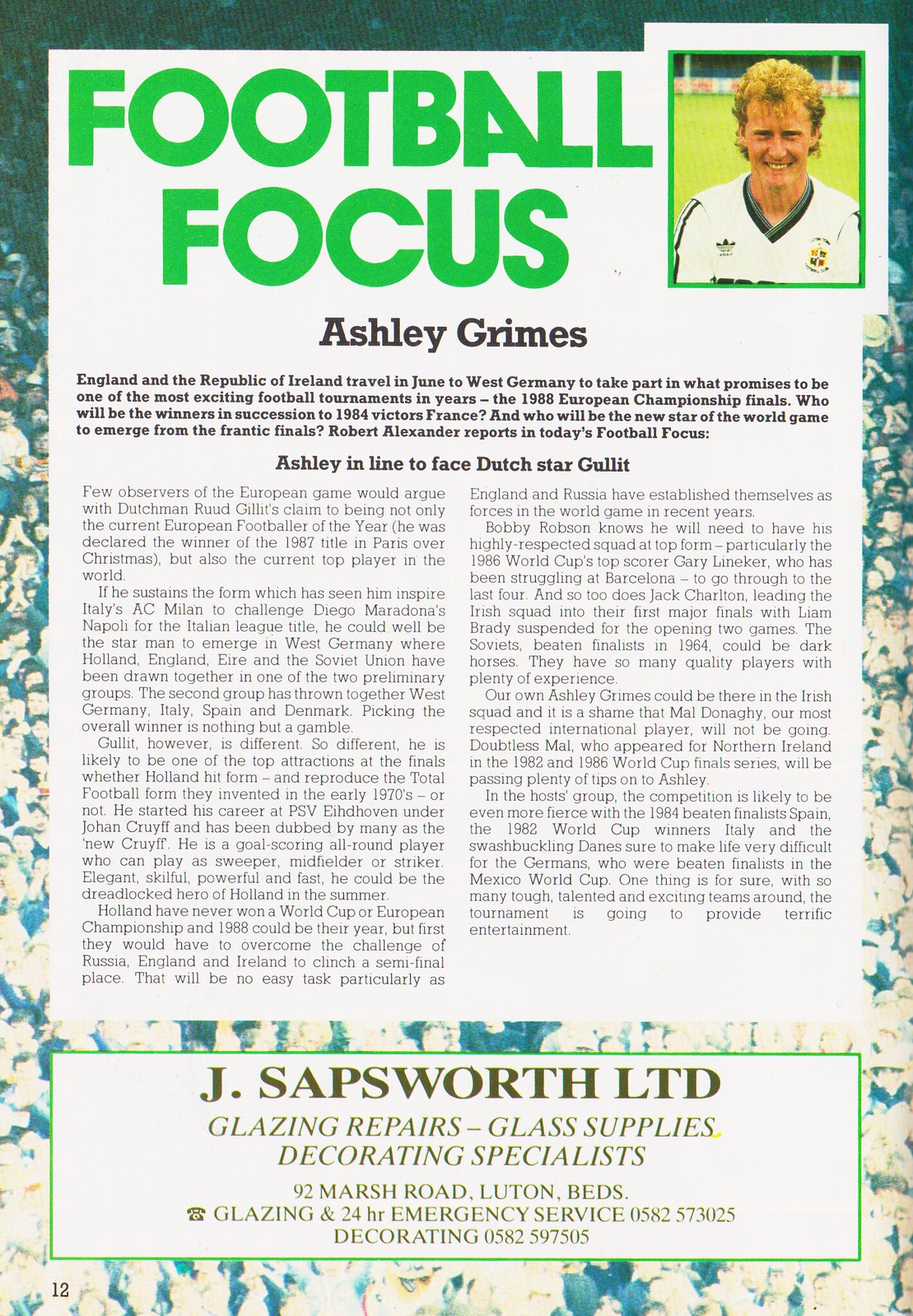The image features a magazine or newspaper article that prominently displays a football focus on Ashley Grimes. At the top, the title "Football Focus" is written in bold green letters, accompanied by a picture of Ashley Grimes in the upper right-hand corner, wearing a red, green, and white jersey. Below the title, her name, Ashley Grimes, is mentioned again in black letters. The article details that England and the Republic of Ireland will travel to West Germany in June to compete in the much-anticipated 1988 European Championship Finals. The piece speculates on which team will succeed the 1984 victors, France, and who might become the new star of the World Game from the finals, with a specific mention of Ashley Grimes being in line to face Dutch star Gullit. The main content is organized into two columns, filled with detailed paragraphs about Ashley’s achievements and unique qualities as a player. At the bottom of the page, marked as page 12, there is a light green-bordered rectangular section dedicated to sponsorship, highlighting J. Sapsworth Limited for glazing repairs, glass supplies, and decorating specialists, along with their contact information.